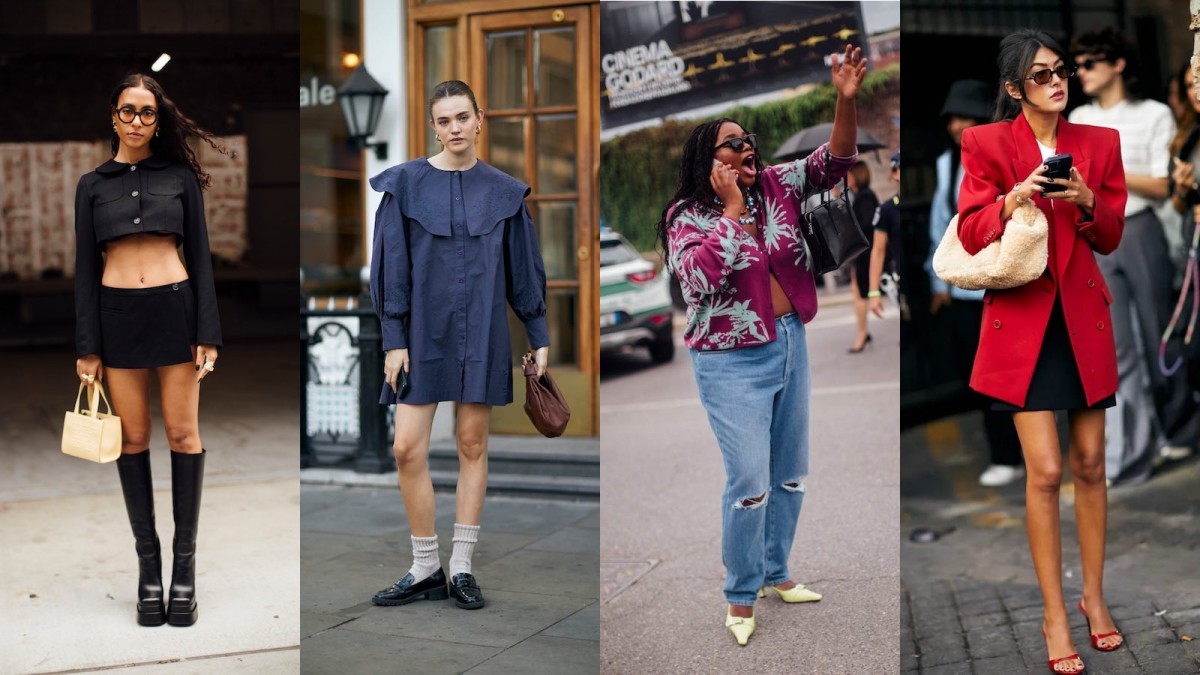This composite image consists of four vertical segments, each portraying a woman standing on different city streets, arranged side-by-side to create a horizontal rectangle. All four photographs are in color and display diverse fashion styles and ethnicities.

Starting from the left, the first woman is a tall, thin, light-skinned African-American, wearing a long-sleeved, cropped black cardigan that reveals her midsection, paired with a very short black skirt. She accessorizes with knee-high black socks, black loafers, and a white beige purse. She's standing on concrete, looking directly at the camera.

The second woman, a Caucasian with black hair, is in front of a wooden door. She wears a very short, navy blue dress with an oversized collar that flares slightly. Her outfit is completed with white ankle socks and black shoes. She holds a brown purse and appears to be posing.

The third woman is an African-American with long hair and dark sunglasses. She has her left arm raised as if hailing a taxi or engaging in a lively conversation on the phone. Her outfit includes a vibrant, burgundy and gray patterned top, blue jeans with holes in the knees, and pointy white heels. Behind her, a sign reads "Cinema Goddard."

The fourth and final woman, likely of Asian descent, wears her black hair in a ponytail and dons dark sunglasses with striking red lipstick. She sports a red blazer with broad shoulders over a black minisk skirt, red open-toe sandals, and carries a large white purse. She appears to be engrossed in her phone.

Each segment varies significantly in style, capturing a unique blend of fashion and cultural diversity.